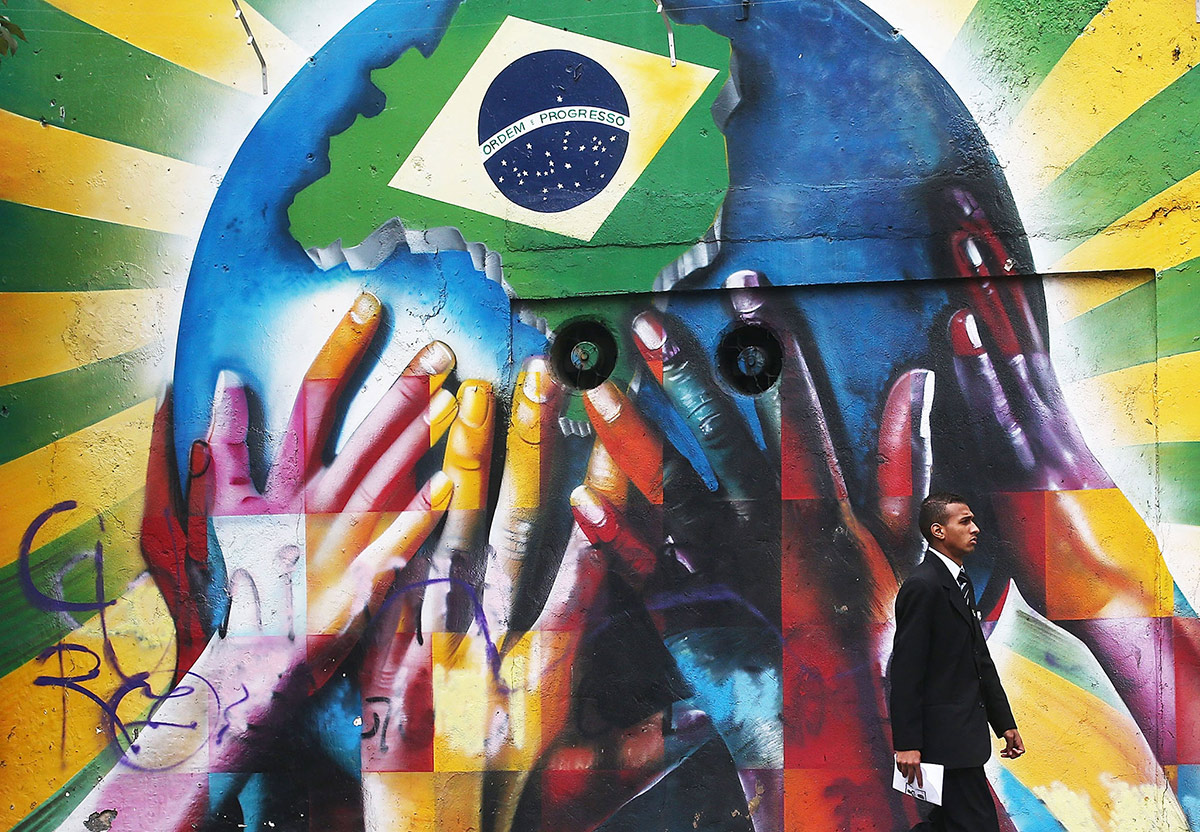This vibrant photographic image captures a moment outdoors, where a young dark-skinned man, likely in his 30s or 40s, strides purposefully in the bottom right-hand corner, depicted in profile, his nose facing right. He is dressed smartly in a black suit paired with a black and white striped tie, clutching a piece of paper in his right hand.

Dominating the background is a striking mural with an elaborate, multicolored design. The mural features a large blue sphere adorned with vibrant imagery, partly flowing off the top of the frame. Encircling the sphere, bands of yellow and green stripes radiate outwards, reminiscent of sun rays.

At the core of the mural, several hands appear to support a globe painted on the blue sphere. Each hand is uniquely colorful: the leftmost hand is purple and yellow; next to it, a predominantly yellow hand; a third hand displays a mix of black, blue, and deep red; and the fourth, to the far right, transitions from red to purple, yellow, and blue. Nestled atop the sphere, the map of Brazil is visible, distinguished by the iconic national flag with the inscription "Ordem e Progresso."

Accentuating the mural are abstract yellow and green stripes that stretch from the sphere to the edges of the frame, blending beautifully. Below the globe, there's text beginning from the bottom left in purple, but it is nearly indiscernible against the vivid backdrop. This interplay of real and painted elements creates a dynamic visual narrative that draws the eye across the entire composition.